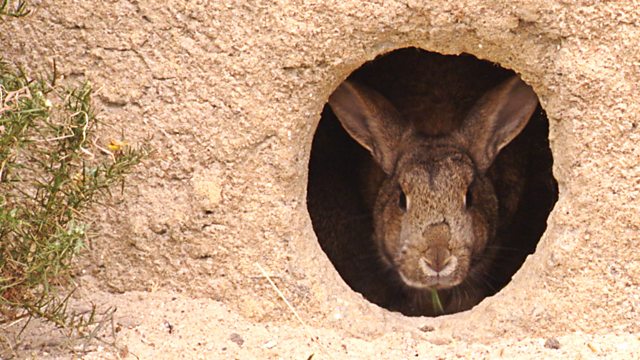The photograph captures the striking image of a brown rabbit peeking out from a large, rough, bumpy hole in a tan, craggy wall or mound of clay and stone. The hole, off-center to the right, occupies most of the image’s height, with only the rabbit's head—its snout, eyes, and perked-up ears—visible. The rabbit holds a bit of green brush in its mouth, adding a touch of color to its predominantly brown fur, which features a light touch of white beneath the nose. To the left of the earthy mound, there is a small, spindly, gray and brown dry brush, emphasizing the desolate and rugged surroundings. At the base of the mound is a layer of sand, providing a subtle contrast in texture and color to the scene.